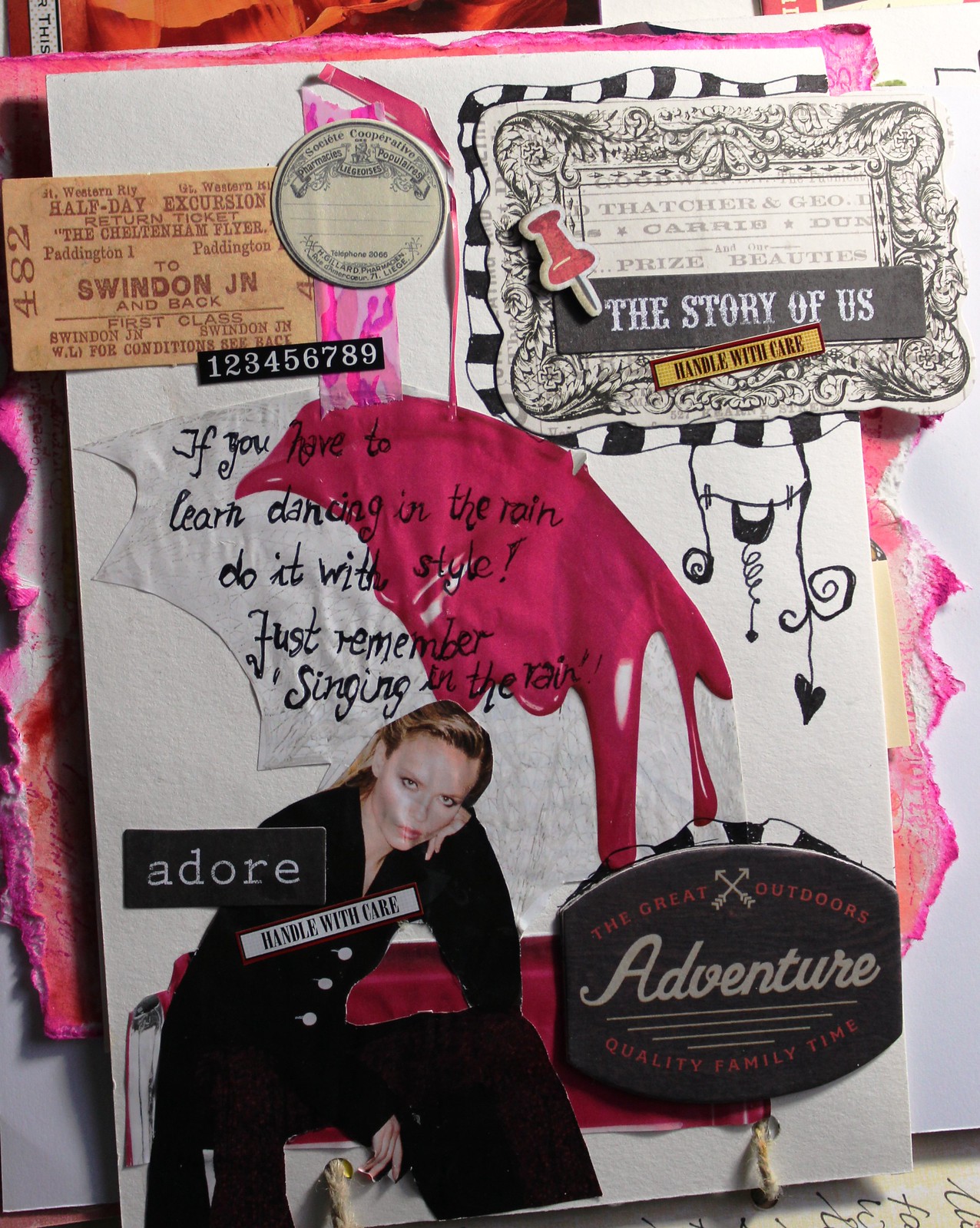In the center of this slightly artistic collage image, a magazine cover dominates the composition. The front cover features an array of visual and textual elements. The top left showcases a ticket labeled "Half Day Excursion on the Cheltenham Flyer, Paddington 1 to Swindon JN and back," indicating a return journey. The top right corner presents a sign reading "The Story of Us, handle with care," adjacent to a red pushpin. Central to the magazine's message, bold text proclaims, "If you have to learn dancing in the rain, do it with style. Just remember Singing in the Rain." Further details include a silhouette of a red bird above this central text. The lower left corner displays an image of a woman seated on a red sofa, dressed in an all-black outfit and posing thoughtfully with her left hand under her chin; over her image, the words "Adore" and "handle with care" are visible. Below her, a black sign with white letters reads, "The Great Outdoors Adventure: Quality Family Time." Splashes of pink paint and other colors like red, orange, black, white, gray, tan, purple, and pink enhance the collage's vivid and dynamic appearance, tying together various items and motifs that seem to reflect personal interests and cherished memories.